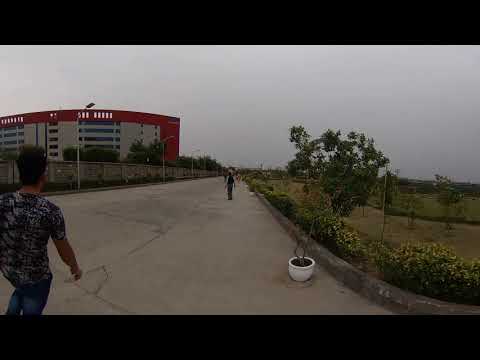In this photograph, taken outside on a cloudy, overcast day, a large building with red siding and long, wide windows stands prominently on the left. The multi-story building features a gray and white exterior, with a tall stone fence separating it from the street. The street itself, which appears worn with cracks, is paved with concrete and is bordered by a paved sidewalk. A man with short black hair, dressed in a black shirt speckled with gray, walks along this street. In the lower left corner, there's another person wearing a blue and white t-shirt and jeans, with brown short hair, walking away from the camera and seemingly engaged with someone in the distance. The sidewalk is lined with green bushes bearing yellow flowers, and near the right side of the image, a white potted plant houses a small green tree. Further ahead, another indistinct figure is visible. The scene is accentuated by patches of grass and distant trees, enhancing the tranquil suburban setting.